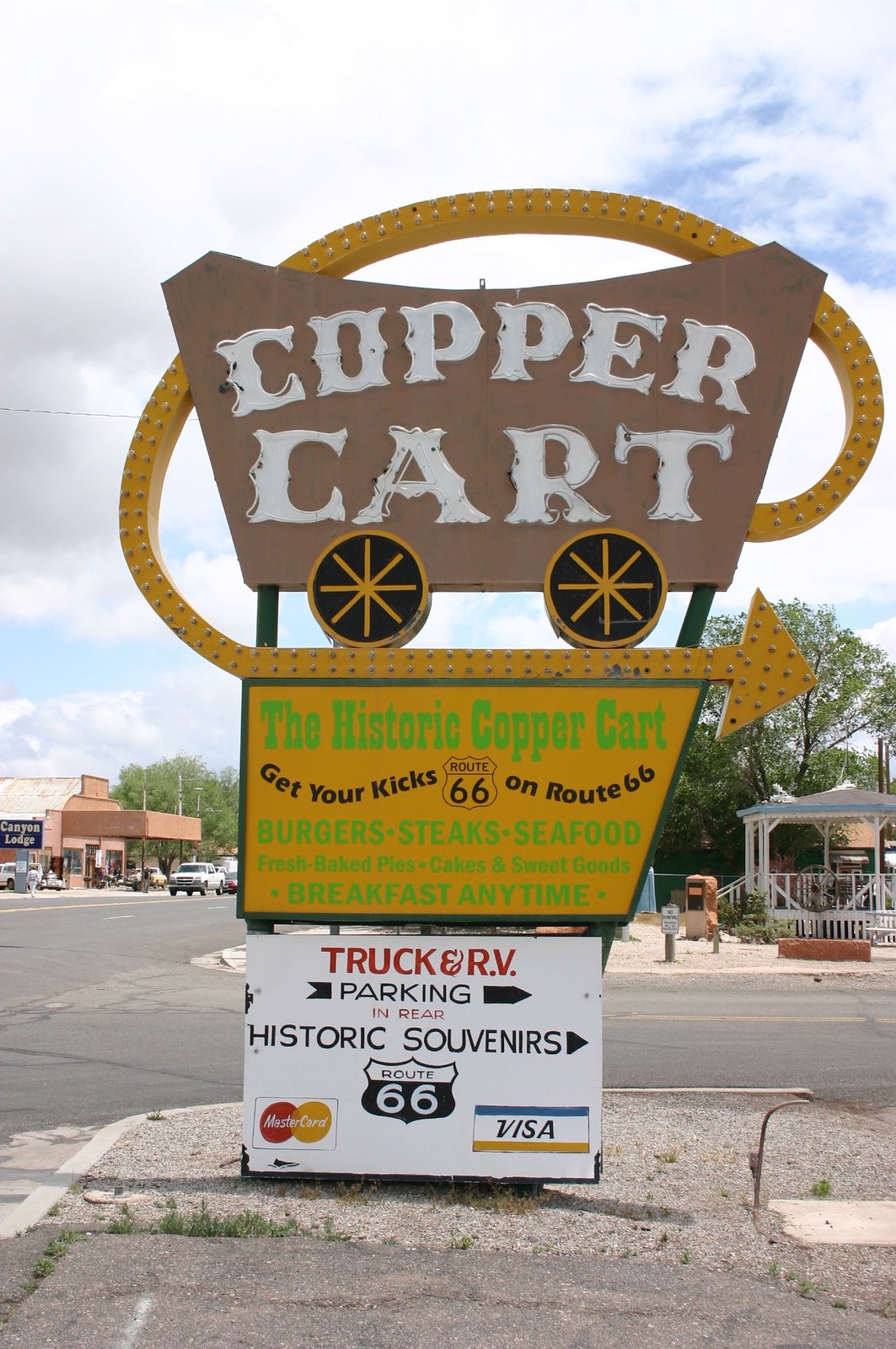In the image, a tall, vintage sign stands prominently at the center of an asphalt multi-lane road. The sign features a rustic, brown covered wagon at the top with the words "Copper Cart" displayed in white across it. Adorning the wagon are golden-colored wheels with intricate yellow spokes. A yellow arrow with light bulbs loops over the wagon, pointing to the right. Below this wagon illustration is a yellow sign with green text reading: "The Historic Copper Cart. Get Your Kicks on Route 66. Burgers, Steaks, Seafood, Fresh Baked Pies, Cakes and Sweet Goods, Breakfast Anytime." Underneath, a white sign states: "Truck and RV Parking in Rear, Historic Souvenirs," flanked by the MasterCard and Visa logos. The backdrop reveals a daytime setting with a cloudy sky, a couple of distant buildings, a pavilion, and some trees. The scene also includes parked cars and a road that intersects near the sign, suggesting the location is outdoors near a restaurant. The sign, likely around 15 to 20 feet tall, embodies a nostalgic charm reminiscent of classic American road trips.